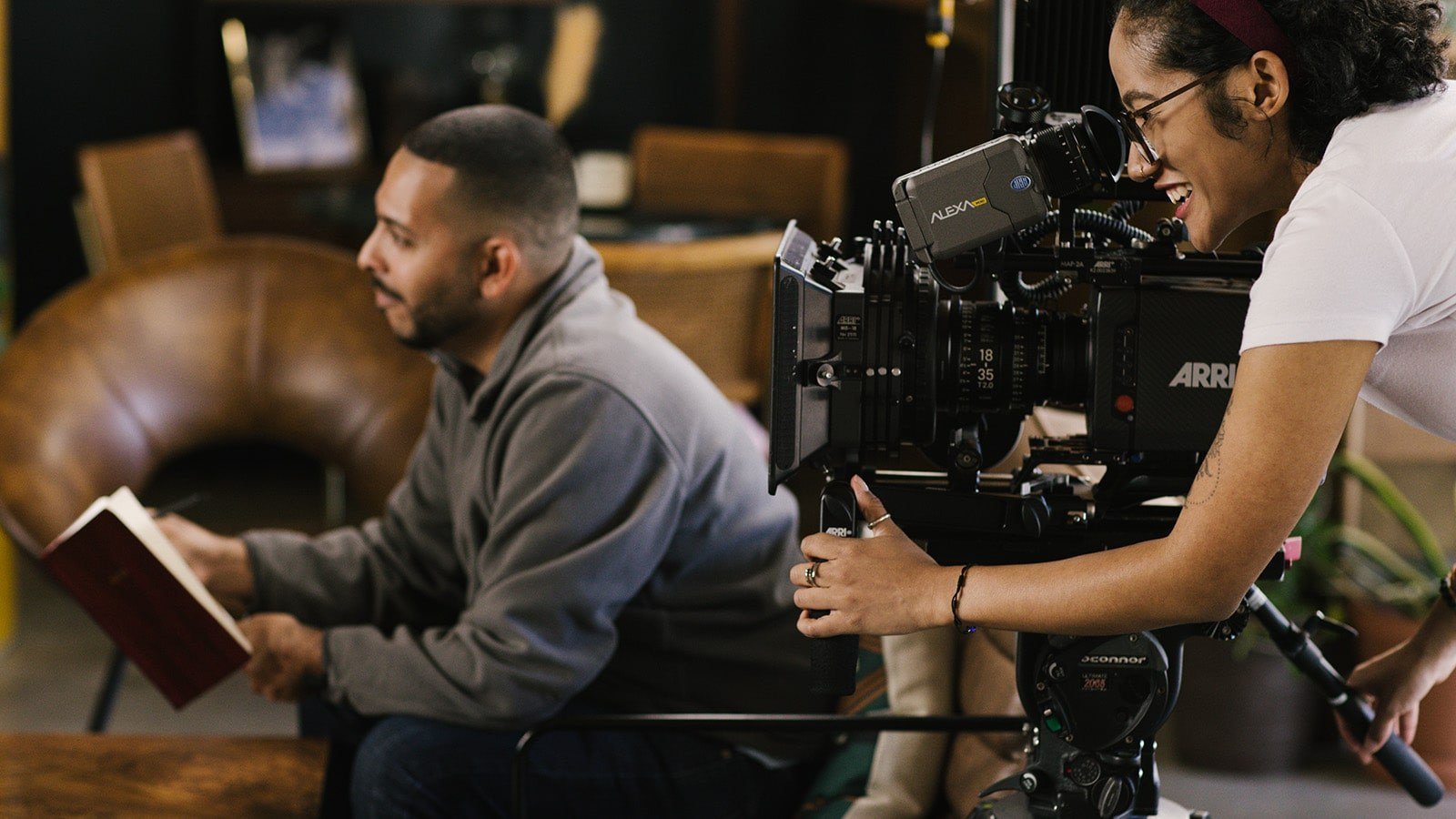This behind-the-scenes image captures a detailed shot of a film set or interview setting. In the foreground to the right, a female camera operator with dark curly hair held back by a burgundy headband, wears a white blouse and focuses on a hefty camera marked "Alexa" on a top attachment. The complex, black camera aligns with production standards, bristling with various components and lettering, including "1835" and other partially obscured details. The camera operator's intent gaze is directed into the lens, further hinting at professional filming.

To the left, a man sits in a chair, facing leftward with a side profile visible. He sports a gray hoodie over blue jeans, and his dark cropped hair complements his tan complexion. The man is engaged with a dark red book featuring beige pages, which he holds in his lap. Notable features include his short mustache and slightly hunched posture, with elbows resting on his knees, capturing a sense of focus or thoughtfulness.

In the background, the set features additional props suggesting an interior room ambiance: tables and chairs, a picture frame on a table, and a distinctive leather bucket chair with croissant-shaped back cushions. Some potted plants can also be spotted near the bottom right, contributing to the scene's everyday realism and detailed depth.